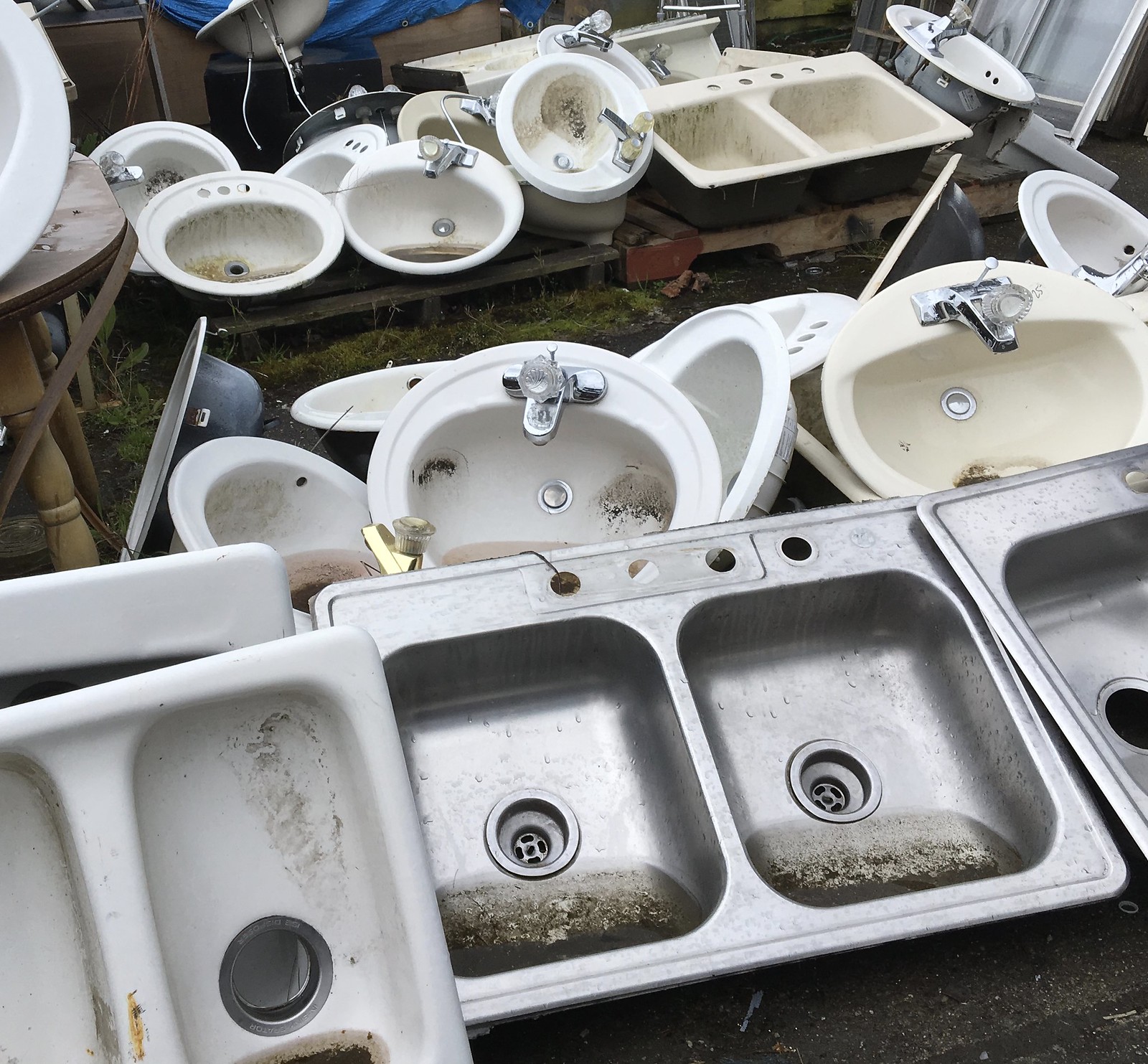This image captures a cluttered outdoor junkyard featuring an assortment of abandoned and used sinks of varying shapes, sizes, and materials. The foreground is dominated by a large two-basin stainless steel sink alongside a double white porcelain sink. Further back, rows of smaller bathroom sinks can be seen, including round ceramic ones and additional commercial-type rectangular sinks. Many of the sinks are partially filled with dirty, stagnant water and show signs of prolonged exposure to outdoor elements, indicated by the presence of algae and soiled interior surfaces. The sinks are organized in several rows, placed directly on the ground and atop wooden pallets. Additional items, possibly parts of a shower assembly and furnishings, are visible in the periphery, including a blue tarp and a table on the left side of the image. Grass growing underneath some pallets further emphasizes the outdoor setting. Overall, the scene suggests an organized collection or disposal area for various types of sinks, possibly within a landfill or a backyard.